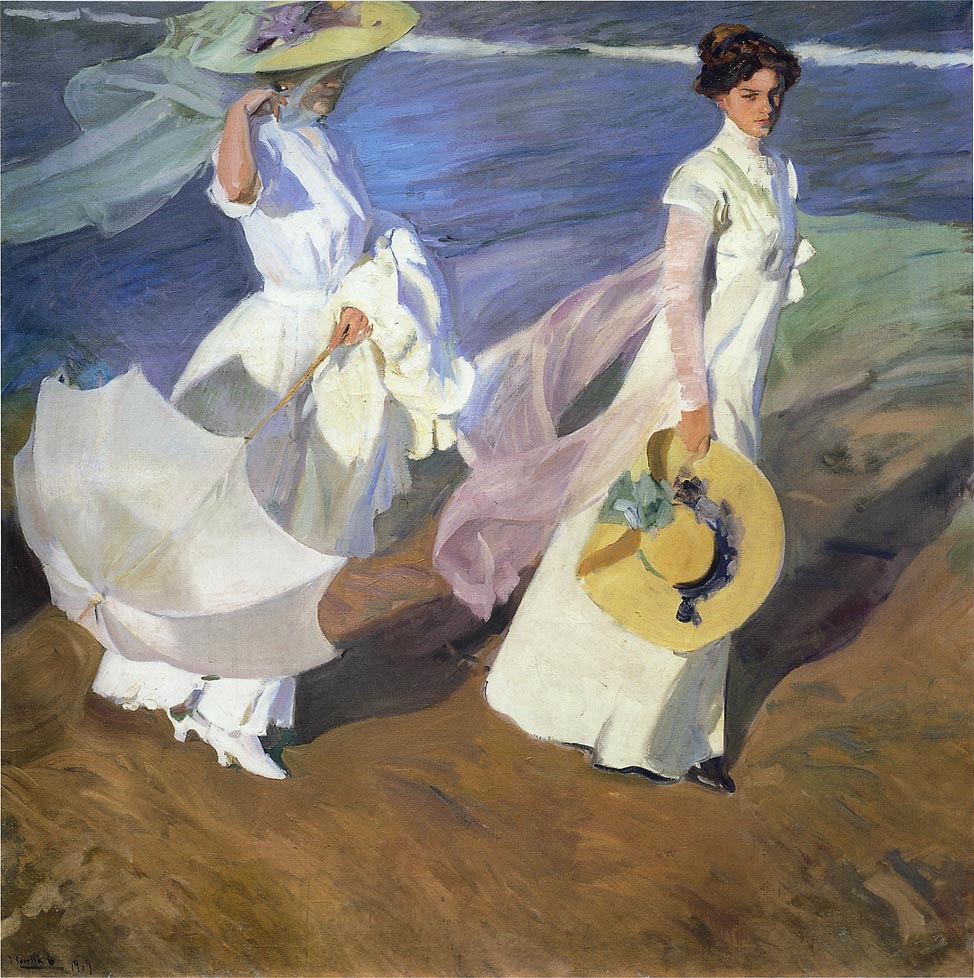The painting "Strolling Along the Seashore" by Joaquin Sorolla, a celebrated piece in the styles of Impressionism and Luminism, showcases two young women walking on a dark brown sand beach with blue waves crashing in the background. Both women are elegantly dressed in long white gowns that reach down to their feet. The woman in front, with brown hair styled in a 1920s fashion, is holding a wide-brimmed straw hat adorned with flowers in her right hand. A pink scarf, reminiscent of cosmos, trails in the breeze behind her. She is wearing dark or black shoes. The woman behind her is distinguished by her large brimmed straw hat with a white veil, which flows gracefully around her face and back. She carries a white parasol in her left hand, which is draped over a white jacket, and she wears white shoes. The serene blue water with its white caps adds a dynamic contrast to the earthy tones of the beach and the overall serene and airy feel of the painting.